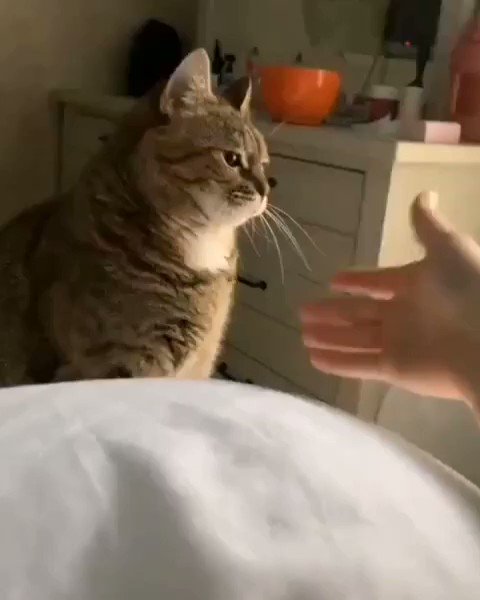In a slightly blurry indoor photograph framed as a vertical rectangle, a tan-colored cat with white fur beneath its chin sits upright on what appears to be a bed, taking up about a third of the left side of the image. With long whiskers and an attentive gaze, the cat stares at a hand reaching out toward it from the right side of the picture. The background suggests a cluttered bedroom, featuring a white cabinet or dresser with black handles and an array of objects on top, including an orange cup and what might be makeup items. The dresser has several drawers, and there's a hint of a large bowl and possibly a lint roller among the scattered items. The overall color palette includes white, off-white, orange, brown, beige, black, and tan, contributing to the cozy yet disorganized atmosphere. The setting, dimly lit, further adds to the intimate and personal feel of the scene.